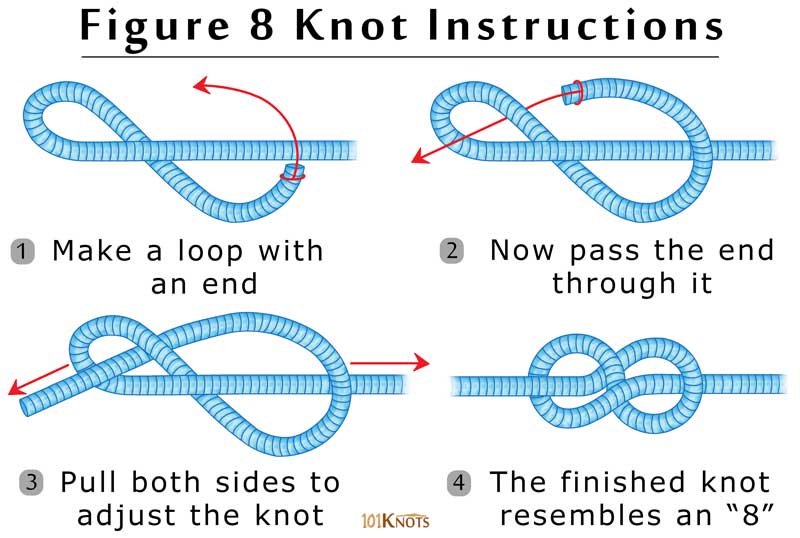The image features detailed step-by-step instructions on how to tie a Figure 8 Knot. At the very top, the title "Figure 8 Knot Instructions" is written in black and underlined against a solid white background. Below the title, the instructions are organized into four numbered steps displayed in a 2x2 grid, each step illustrated with a blue rope and red directional arrows. 

1. The first image, located in the upper left corner, shows a horizontal blue rope forming part of a Figure 8 with a red arrow indicating how to complete the step. The caption reads, "Make a loop with an end."
2. The second image, in the upper right corner, continues from the first step, showing the blue rope with the bottom part brought up further to almost complete the Figure 8. The caption reads, "Now pass the end through it."
3. The third image, in the lower left corner, depicts pulling both sides of the rope to adjust the knot, with red arrows emphasizing the motion. The caption reads, "Pull both sides to adjust the knot."
4. The final image, in the lower right corner, shows the completed knot resembling a figure eight. The caption reads, "The finished knot resembles an eight" (in parentheses). 

Additionally, the bottom of the image includes the text "101 knots" written in gold.